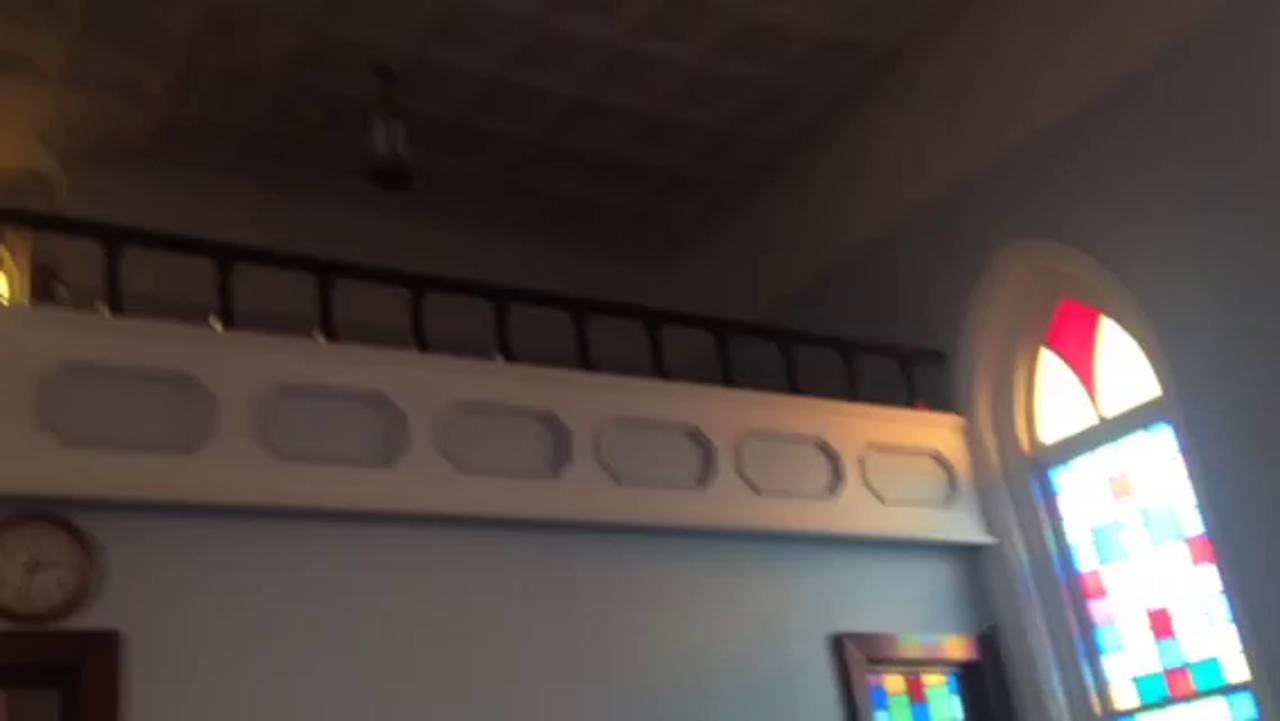This somewhat blurry photograph captures the interior of a dimly lit church from an awkward, upward angle, suggesting it may have been taken hastily. Dominating the image is a stained glass window nestled in an archway. The main window comprises predominantly square panels in hues of green, yellow, white, and red, with cone-shaped glass sections crowning the top within the arch. To the right of the window are glimpses of additional stained glass panels, featuring similar square segments in red and blue. The shot also reveals architectural details: a black railing running horizontally near the height of the window, white and wood trim framing parts of the scene, and light blue paint on the walls. The lofty ceiling exhibits a checkered pattern, and a lantern or light fixture hangs from above. On the left side of the image, there's a clock positioned above what appears to be a picture or frame, accompanied by geometric shapes and a balcony section higher up, although the doorway isn't fully visible. A soft, yellowish light emanates from the top left corner, enhancing the church's serene ambiance.